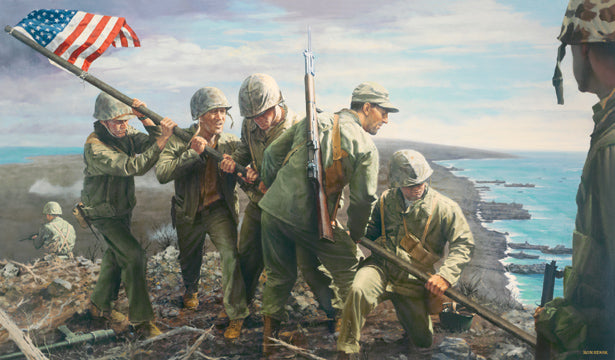In this horizontally aligned, rectangular image that bears a striking resemblance to a painting or CGI illustration, seven soldiers are depicted in a scene reminiscent of a battlefield. The focal point is the five soldiers in the center who are laboriously raising a long wooden pole carrying an American flag, which is positioned in the upper left-hand corner of the image. Each soldier is adorned in military clothing, with helmets except for one soldier who wears a cap. The soldier in the very center, who has his back turned to the viewer, is identifiable by the rifle strapped to his back. To the left, one soldier grips the pole while facing right. Adjacent to him, another soldier stands with both hands on the pole, his head slightly turned. Continuing to the right, a third soldier mirrors the same grip and stance. Next, a soldier, facing mostly away from the viewer and with a rifle on his back, also holds the pole. Beside him, a kneeling soldier has his left hand on the pole with his head turned slightly. At the bottom right corner of the image, a partially visible soldier stands, observing the flag-raising efforts of his comrades, facing left and away from the viewer. In the far background on the right side, there is a hint of a shoreline with a blend of blue and white water, juxtaposed against a cloudy sky of mixed white, gray, and blue hues. To the left, another soldier sits, further adding depth to this evocative and detailed scene.